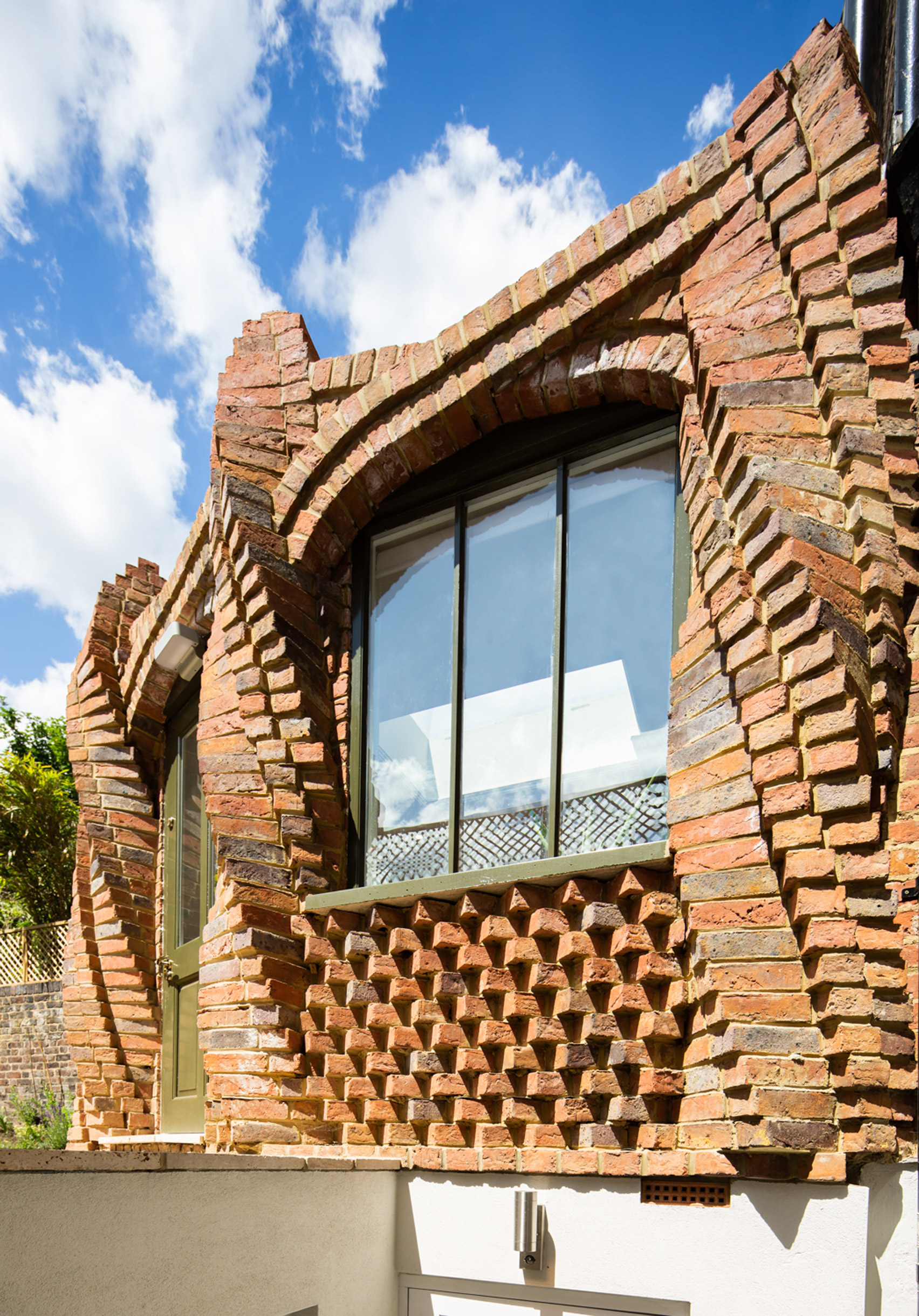This vertically aligned rectangular photograph captures the intricate façade of a building made from a mix of rust-colored and soft gray bricks. The image showcases a large, floor-to-ceiling window consisting of three vertical panes aligned side by side, creating an impressive central feature. Surrounding the window, the bricks are artfully arranged in a decorative and dynamic manner, giving a sense of movement and flow. They are placed horizontally across the top and twist down the sides, simulating a winding staircase pattern, and at the bottom, the bricks are staggered, revealing their ends and creating an engaging geometric design. 

To the lower left, a different shade of brownstone forms a large retaining wall, crowned with a lattice wood fence, adding more texture to the scene. The background includes trees behind this wall, augmenting the natural setting. The upper part of the photograph is dominated by a crisp, clear blue sky with feathery white clouds, lending a serene and airy atmosphere to the overall image.